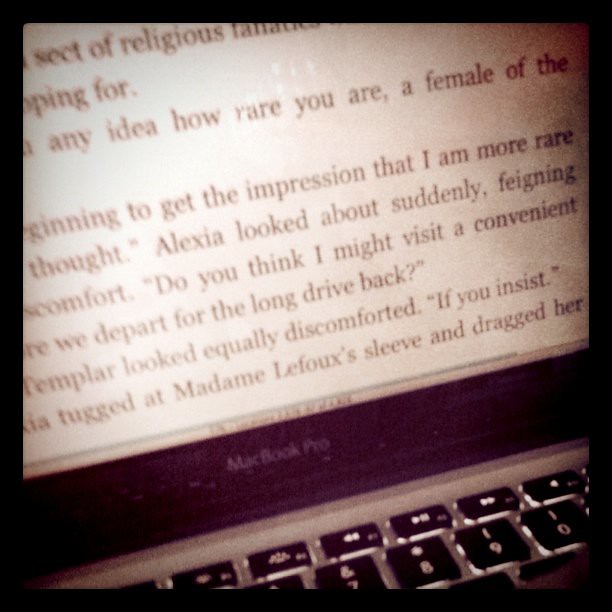The image depicts a blurry and grainy close-up photograph taken at night of a MacBook Pro screen and keyboard. The photograph appears to be an old Instagram photo with a filter applied. The screen is partially visible and contains text in a Times New Roman font, possibly displayed in Microsoft Word or Apple's Pages application. The visible portion of the text reads: "sect of religious fanatics probably hoping for. Any idea how rare you are, a female of the beginning to get the impression that I'm more rare, thought Alexia looked about, suddenly feigning discomfort. Do you think I might visit a convenient—where we depart for the long drive back? Templar looked equally discomforted. If you insist, some kya tongue that Madame LeFou sleeved and dragged her." The screen has a big black border with rounded corners, and the image captures part of the MacBook Pro's keyboard, showing the backlighting and keys such as the play button, sound controls, and a portion of the number row including the numbers 7, 8, 9, and 0.